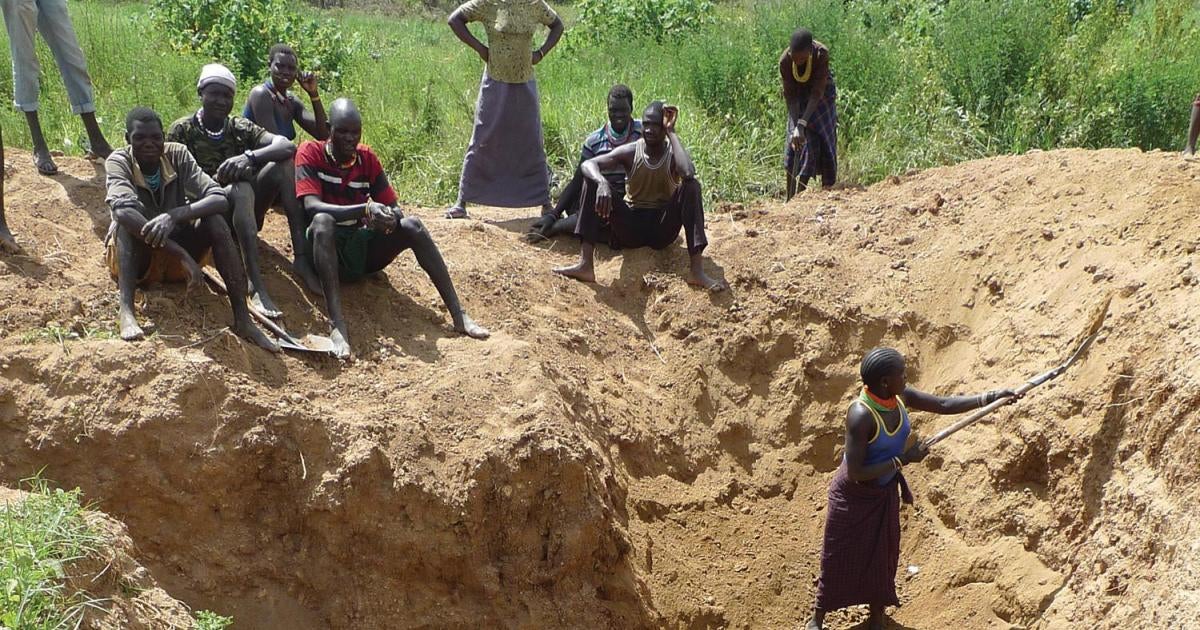In this outdoor daytime photograph set in an African country, a group of approximately 11 to 12 people is seen around a large, deep hole they have dug in the light, sandy dirt. The foreground prominently features a woman with tightly braided hair, dressed in a blue tank top trimmed with yellow, a long dark purple skirt, and a green and orange handkerchief around her neck, actively digging with a long stick or shovel. Above her at the edge of the hole, there are several individuals, primarily young men, sitting and taking a break. Notably, one man in the group wears a white hat. To the left, a woman stands with her fists on her hips, dressed in a long blue skirt and a yellow short-sleeved shirt with flowers. The background shows tall grass, indicating a semi-rural setting. Most of the people are barefoot and sporadically looking towards the camera, suggesting a brief pause from their work.